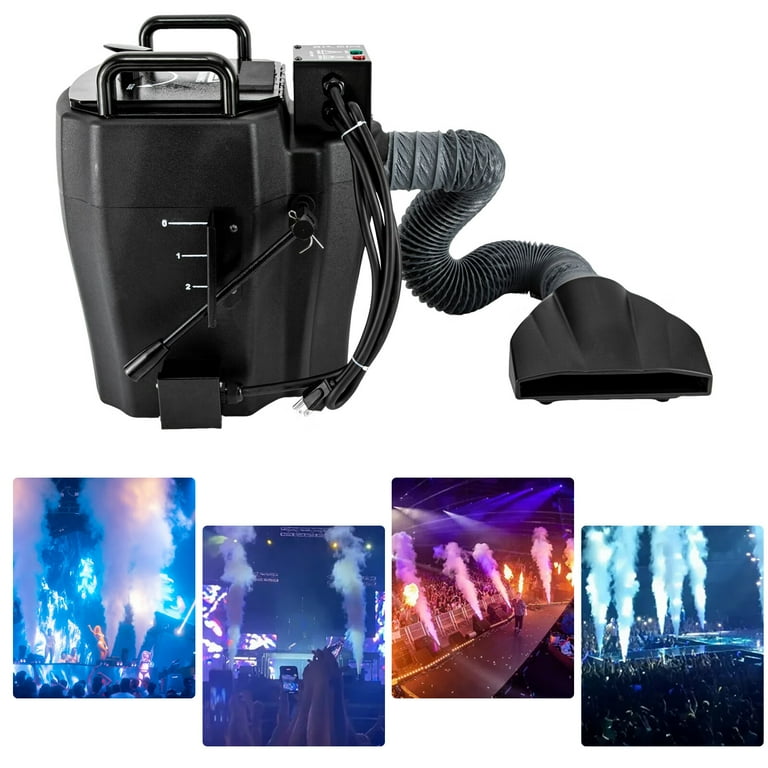The image is a color photograph that appears to serve as an advertisement for a fog machine typically used in club settings. At the top of the image is a black machine with two handles and a hose, reminiscent of a vacuum cleaner. The device features a plug, an outlet for releasing fog, and fill lines on its side. Additionally, it has a red and green button on top. Below it, there are four smaller images showing the fog machine in action during live performances. The first smaller image has a blue hue with white smoke plumes, the second is set against a darker blue background, the third features vibrant fire-like colors such as purple, pink, orange, and yellow, and the fourth returns to a blue theme with plumes of smoke going straight up. In these images, you can see performers on stage, the crowd, and the dramatic effect of the tall plumes of white smoke being emitted by the machine.